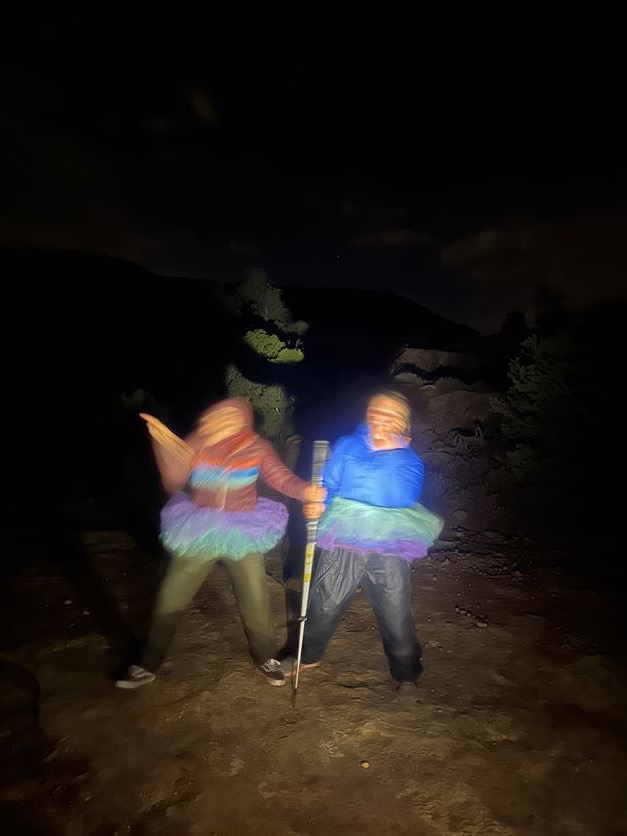In this blurry photograph, two children are the focal point, both dressed in colorful tutus. The background is completely black, providing a stark contrast to the lit figures of the children who stand on what appears to be dirt or mud. On the right, a child is seen wearing a blue jacket paired with a green and purple tutu, black pants, and tennis shoes. The child on the left is dressed in an orange jacket, green pants, black tennis shoes, and an identical tutu to the child on the right. Due to the blurriness, their faces are indistinguishable, making it hard to determine their genders. The predominant hues in this image include blacks and browns from the background and ground, while the children’s attire features vibrant greens, blues, oranges, and purples.